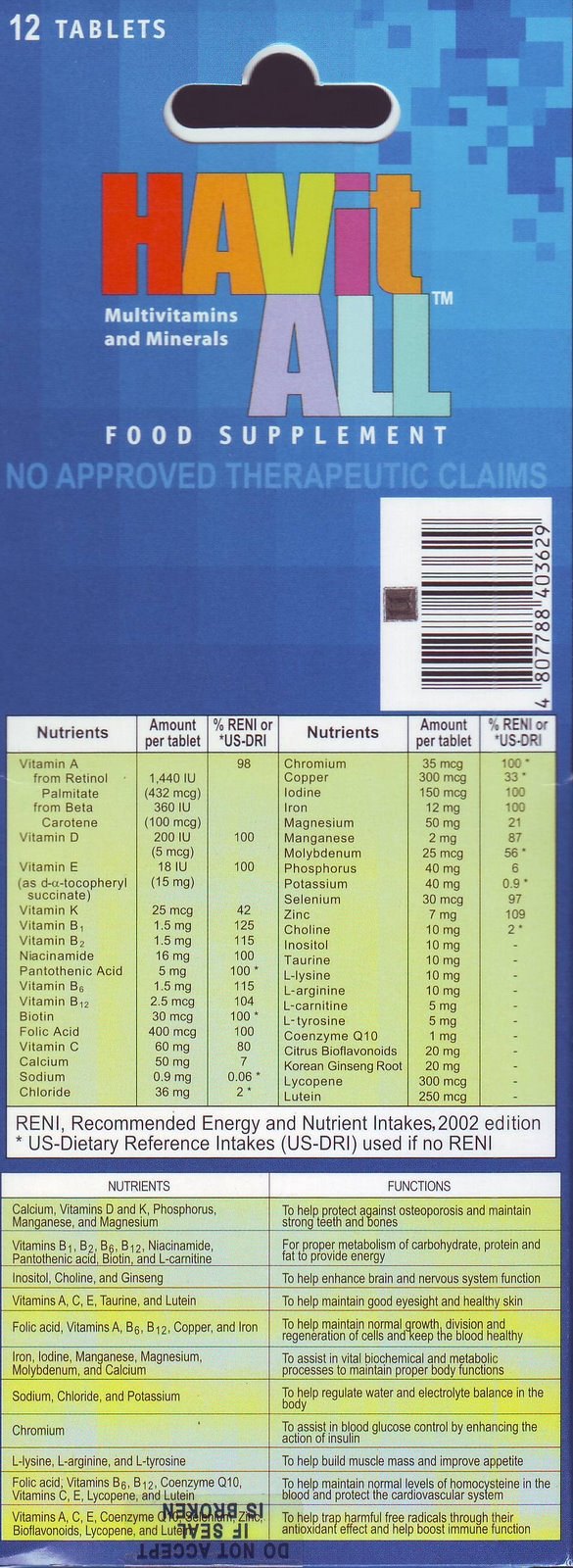The image displays the packaging of a food supplement named "Habit All," which contains 12 tablets. The package has a tall rectangular shape and a blue background with a pattern of small squares that get lighter towards the top. "Habit All" is prominently featured on the top left, spelled as "H-A-V-I-T" on the first line in multicolored letters—red, orange, yellow, purple, and orange—and "ALL" in lavender and light blue letters on the line below. Beneath the product name, the text "No approved therapeutic claims" is displayed. The barcode is situated on the top half of the package. The bottom half of the package is a yellow rectangle listing all the nutrients and their functions. These nutrients include vitamins A, D, E, K, various B vitamins, niacinamide, folic acid, biotin, vitamin C, calcium, sodium, chloride, and iodine (150 micrograms). The nutritional information highlights the benefits such as protection against osteoporosis, strong bones, proper metabolism, brain and nervous system function, good eyesight, healthy skin, maintenance of normal blood homocysteine levels, and antioxidant properties to help trap harmful free radicals.